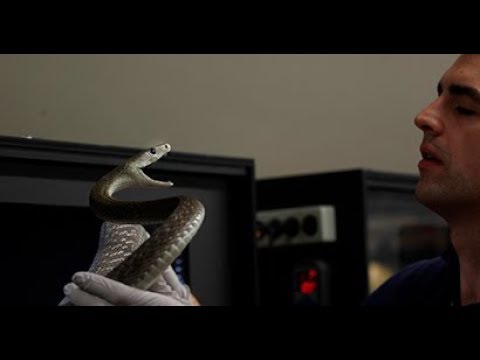In this detailed color photograph, a white man with dark eyebrows and beige skin is positioned on the right side, attentively handling a snake in his left hand, which is protected by a gray latex glove. The snake, which appears to be a gray-colored viper, is poised as though it is about to strike, with its mouth wide open displaying no visible fangs. Its skin features distinct patterns, and its black eye and nostril are clearly visible. The background features a series of illuminated terrarium-like incubators that appear to house various snakes, some equipped with electrical dials and red lights. A yellowish triangle and other controls suggest a temperature-regulated environment. The setting is likely a controlled space designed for the care and study of snakes, with brown walls providing a neutral backdrop to the scientific scene. The man seems to be carefully examining the snake, possibly having just taken it out of its enclosure for closer inspection.